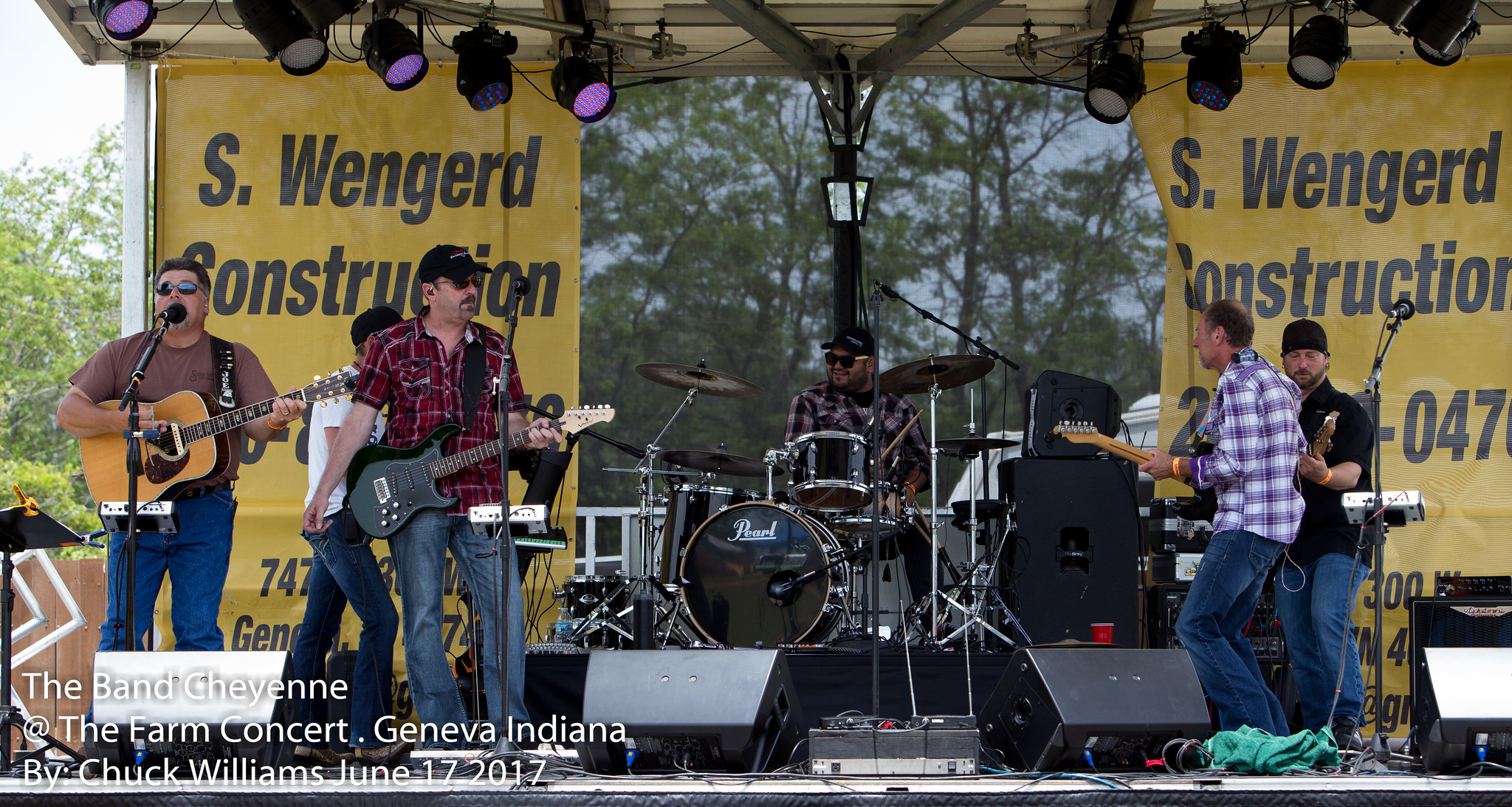The image depicts a vibrant performance by the band Cheyenne at the Farm Concert in Geneva, Indiana, on June 17, 2017, captured by photographer Chuck Williams. The stage is alive with energy as five musicians, mostly middle-aged men, dominate the scene. The two electric guitarists, both sporting checkered shirts, flank either side of the stage along with the drummer, who is also adorned in a checkered shirt and seated centrally behind an extensive drum set. The bassist, distinguishable in a black t-shirt, anchors the rhythm section, while the acoustic guitarist and vocalist, wearing a brown t-shirt, stands to the left. Most of the band members are wearing sunglasses, adding a cool vibe to the performance. A sound system surrounds them, indicating a well-equipped setup. Additionally, a yellow banner with black text for S. Wengard Construction displays prominently on the left and right sides of the stage. The lower left corner of the image features the photo credits, providing clear attribution and contextual details.